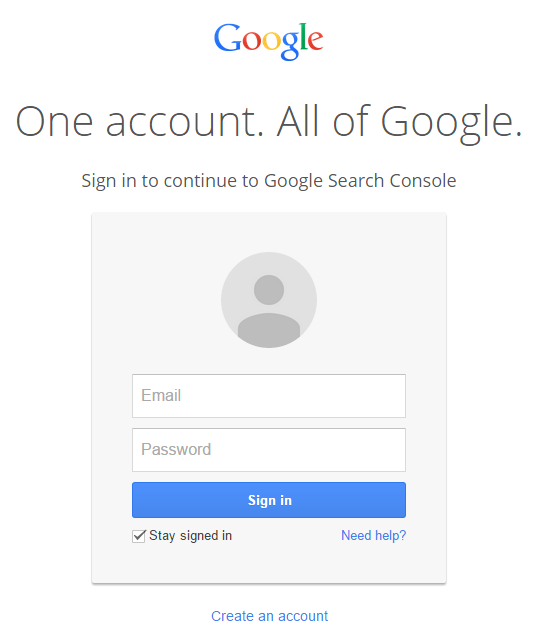Screenshot of the Google Sign-In Page for Google Search Console:

The image is a screenshot of the Google Sign-In page specifically for accessing Google Search Console. At the top of the page, the Google logo is displayed prominently in its signature multicolored design (blue, red, yellow, and green). Beneath this logo is the tagline "One account. All of Google," followed by the instruction, "Sign in to continue to Google Search Console."

The primary section of the page consists of a gray rectangle and an abstract 3D figure representing a generic user profile. Below this, there are text fields labeled "Email" and "Password," accompanied by a blue "Sign In" button featuring white text.

Additional options include a checkbox labeled "Stay signed in," which is pre-checked, and a hyperlink "Need help?" marked with a question mark for user assistance. Toward the bottom of the page, ample white space provides a clean layout, and another hyperlink, "Create an account," is presented in blue text, inviting new users to register.